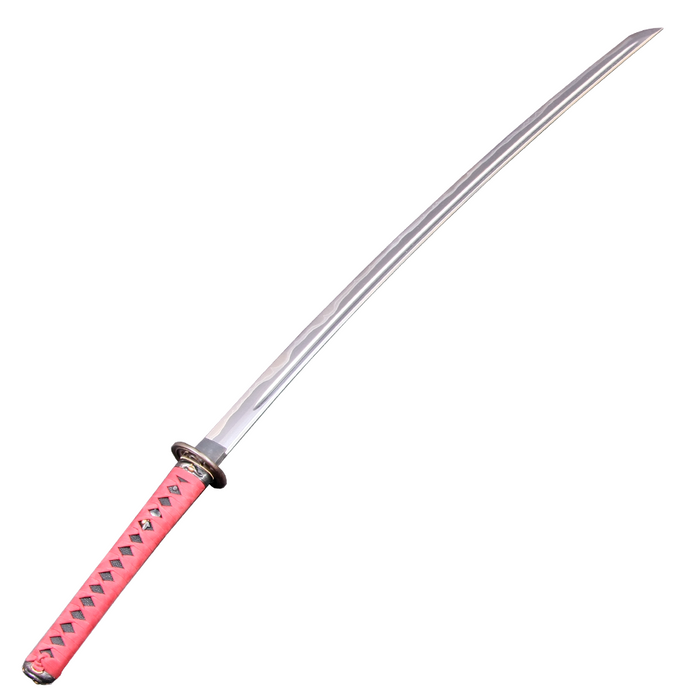This image features a detailed depiction of a Japanese katana set against a solid white background. The katana is oriented diagonally, with the handle positioned in the lower left corner and the blade extending to the upper right. The hilt of the katana is wrapped in a dark pink covering with a diamond-shaped cutout, revealing the black or very dark gray handle beneath. There is a silver tip visible under this wrapping. Above the hilt, before the blade starts, is a circular cross-guard (tsuba) that appears to be a brownish-gold or dark brass color.

The blade itself is long and silver, featuring a pointed tip. It is distinguished by its sharp edge on the left side, which is finely ground to create a few smooth waves. The blade is further detailed with a vertical groove, known as a bo-hi, running along its length. Despite its inherent metallic sheen, the blade also displays some faint white streaks, which may resemble paint but are uncertain. This artistic depiction showcases the katana's craftsmanship and elegance without any text or border to distract from its form and details.